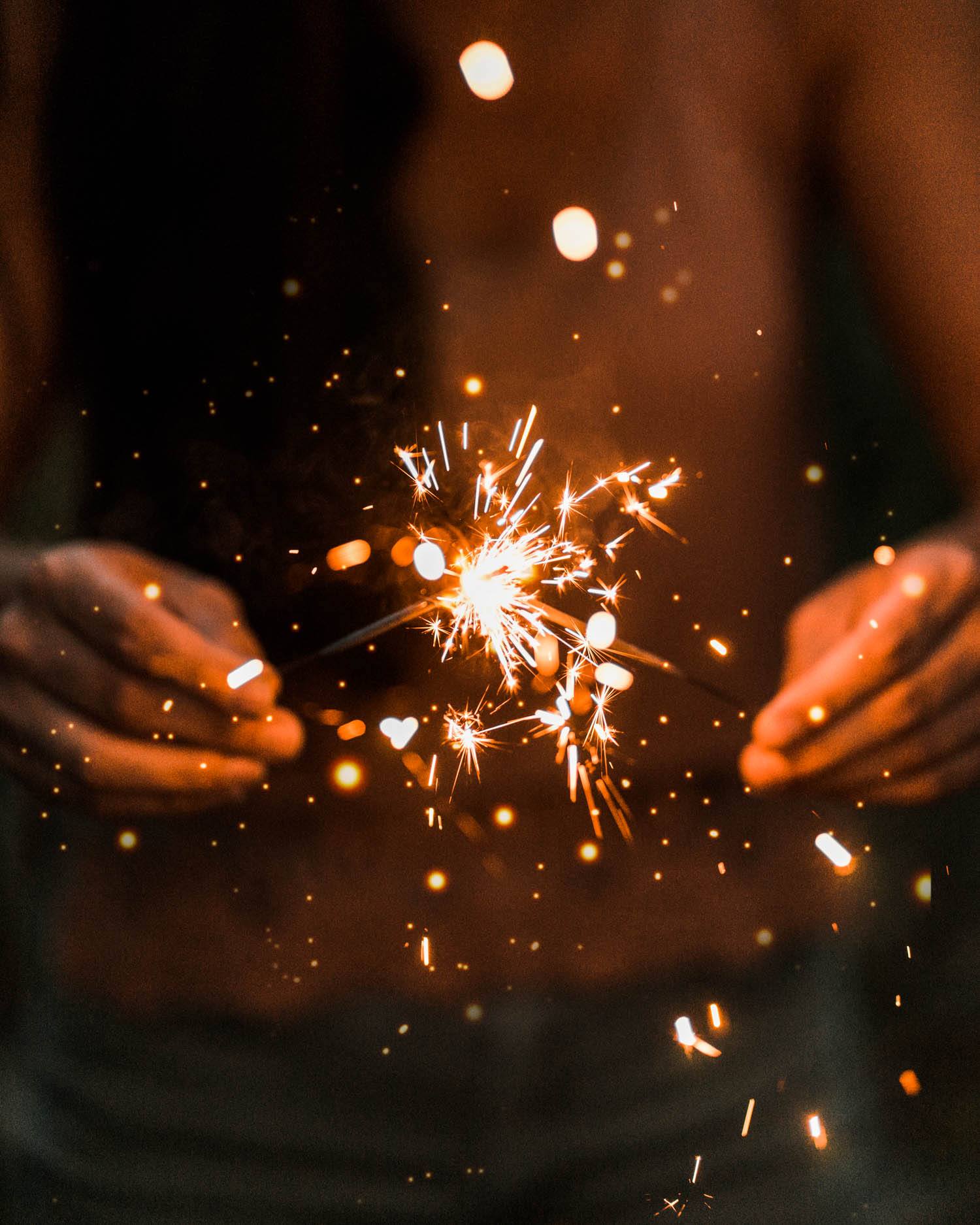In this evocative, vertical portrait, two hands—identifiably dark brown and likely belonging to a Black or African-American individual—are seen holding two slender sparklers that meet in the center of the image, creating a burst of brilliant, orange flame. The sparklers erupt in a dazzling display of light and sparks, illuminating the scene against a rich, chocolate-brown backdrop that suggests it was captured in darkness. The fiery spectacle produces white and orange streaks and specks, lending a festive and celebratory atmosphere to the entire composition. Slight apparitions of the person holding the sparklers—revealing hints of jeans, a shirt, an arm, and a shoulder—emerge subtly through the glittering pyrotechnics, adding depth and human presence to the joyful moment.